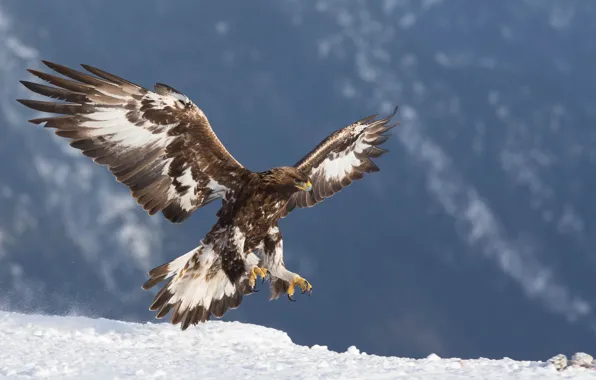This is a beautifully detailed nature photograph depicting a large raptor bird, possibly an eagle or hawk, in the midst of landing on a snowy terrain. Captured in a horizontal, rectangular orientation, the raptor stands out magnificently against a bright blue sky adorned with thin, white cirrus clouds. The bird, exhibiting predominant brown feathers with patches of white on the inner parts of its wings and tail, is facing right with its wings fully outspread and its yellow talons poised beneath its body. Its head is crowned with brown feathers, and it has a distinct yellow, curved beak typical of raptors. The foreground of the image features a pristine, snow-covered ground, while the backdrop, although slightly blurred, hints at a dark gray mountainside intermittently streaked with snow. The horizon line is positioned low, encompassing the lower quarter of the photograph, accentuating the vivid daytime ambiance of the natural setting.